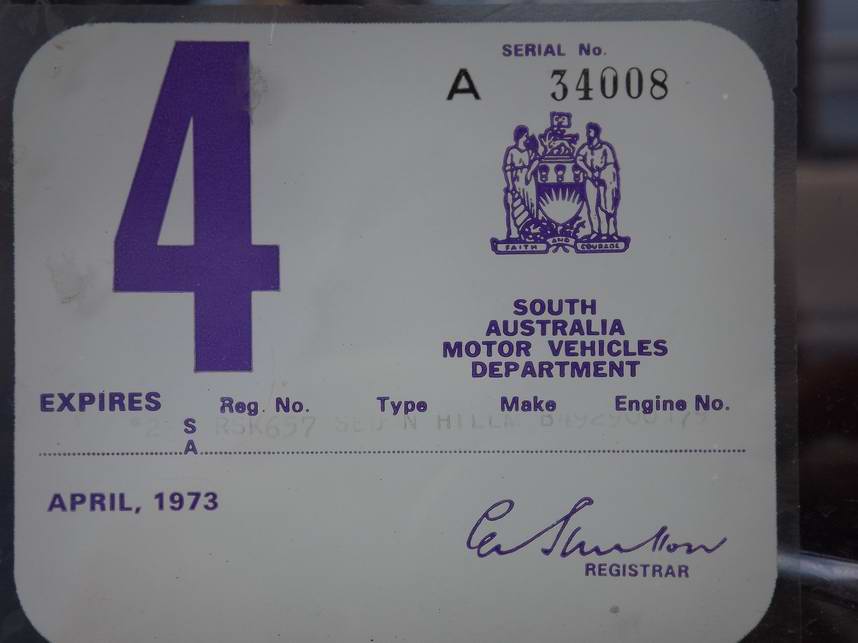This photograph displays a vintage, square-shaped piece of paper with rounded edges, resembling an old-timey driver's license from South Australia. The card predominantly features a purple and white color scheme. Prominently displayed on the top left is a large purple number "4". Adjacent to it is a detailed serial number "A 34008" in dark lettering. The document is issued by the South Australia Motor Vehicles Department and bears the expiration date of April 1973. 

Central to the card is a logo depicting two Greek figures standing in front of a hearth with a ribbon bearing the words "Faith and Courage," which likely symbolizes an Australian emblem. Further down, the registration number "RSK657" is visible, though other specific vehicle details such as type and make are partially illegible. The card also includes fields for additional vehicle information like the engine number, which are represented by a series of dots. A signature from the registrar is present but unreadable. The document is meticulously arranged with labels and information, providing a glimpse into the vehicle registration practices of historical South Australia.